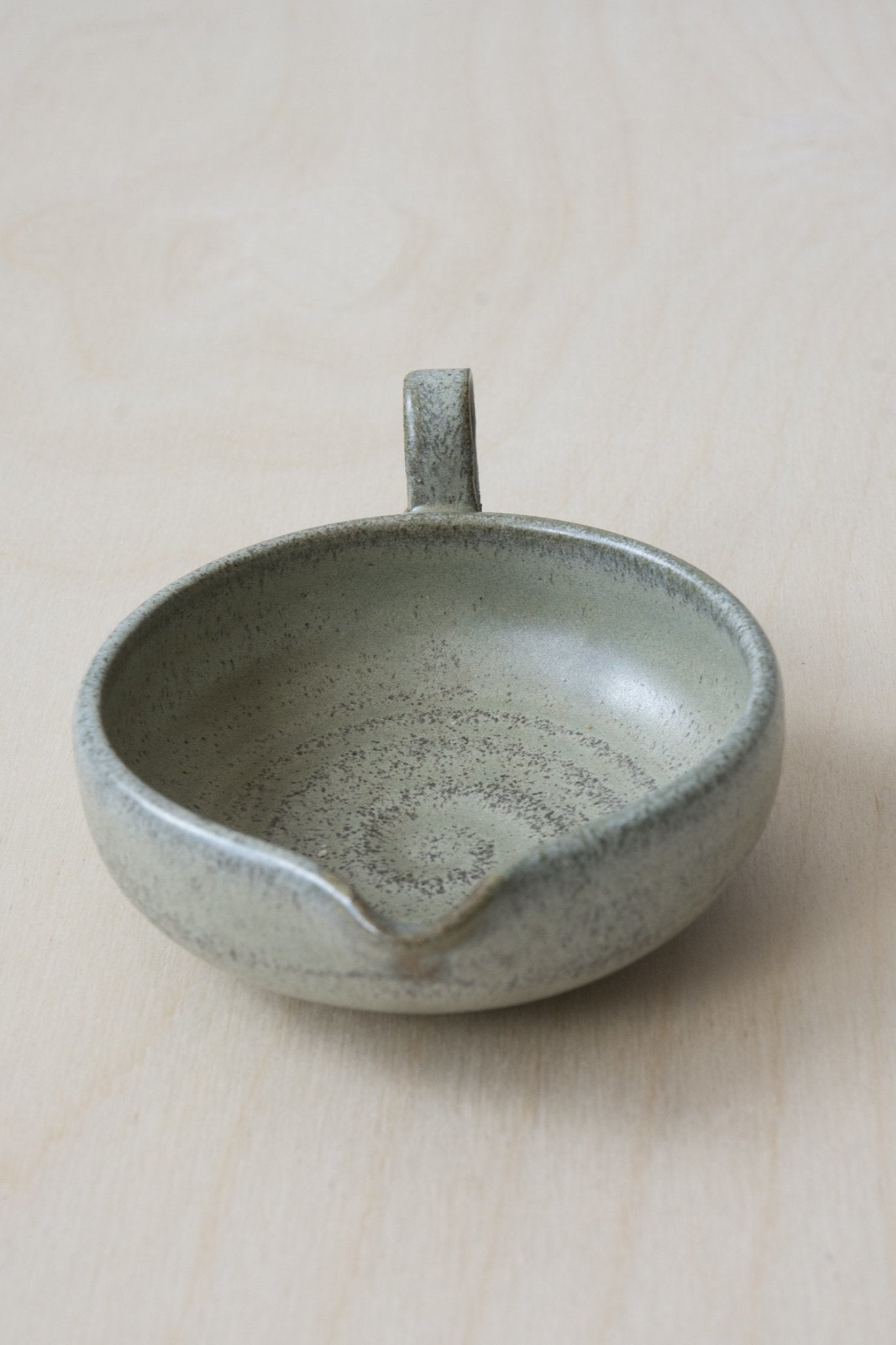This image features a small, polished piece of pottery sitting on a light, whitewashed wooden surface. The pottery is predominantly gray, with different hues and dark speckled circles creating a subtle pattern across its smooth exterior. The vessel is circular with a curved spout designed for pouring liquids, making it resemble a gravy or syrup boat. The rim stands about an inch above the base, and though partially obscured, a looping handle can be seen at the back, indicating its functionality as a carrying vessel for tabletop use. The wood surface, likely a table, is finely grained, with light brown tones that contribute to an overall indoor setting. The pottery’s shadow is cast towards the right, enhancing the image's depth and texture.